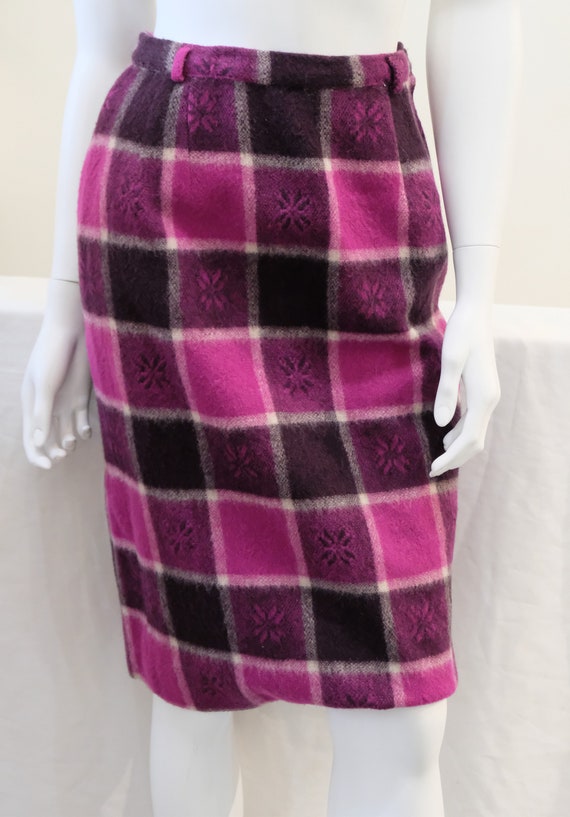This image features a white plastic mannequin, delicately poised and cut off just above the waist at the top and just below the knees at the bottom. The mannequin's thin arms are visible from the elbows down, with one arm slightly more prominent as it is turned a bit to the left, revealing more of its left arm. The mannequin is wearing a plaid skirt with a fitted waist and several belt loops. The skirt, which falls to just above the knees, showcases a vibrant pattern of deep pink, magenta, and various shades of purple with black squares, all interspersed with white lines. Within some of the darker squares, there is an intricate floral design composed of paired petal-like images, adding an extra touch of detail. The backdrop is a blend of gray and tan, providing a neutral contrast to the vivid colors of the skirt. The mannequin's hands hover gracefully over the skirt, accentuating both its texture and complexity.